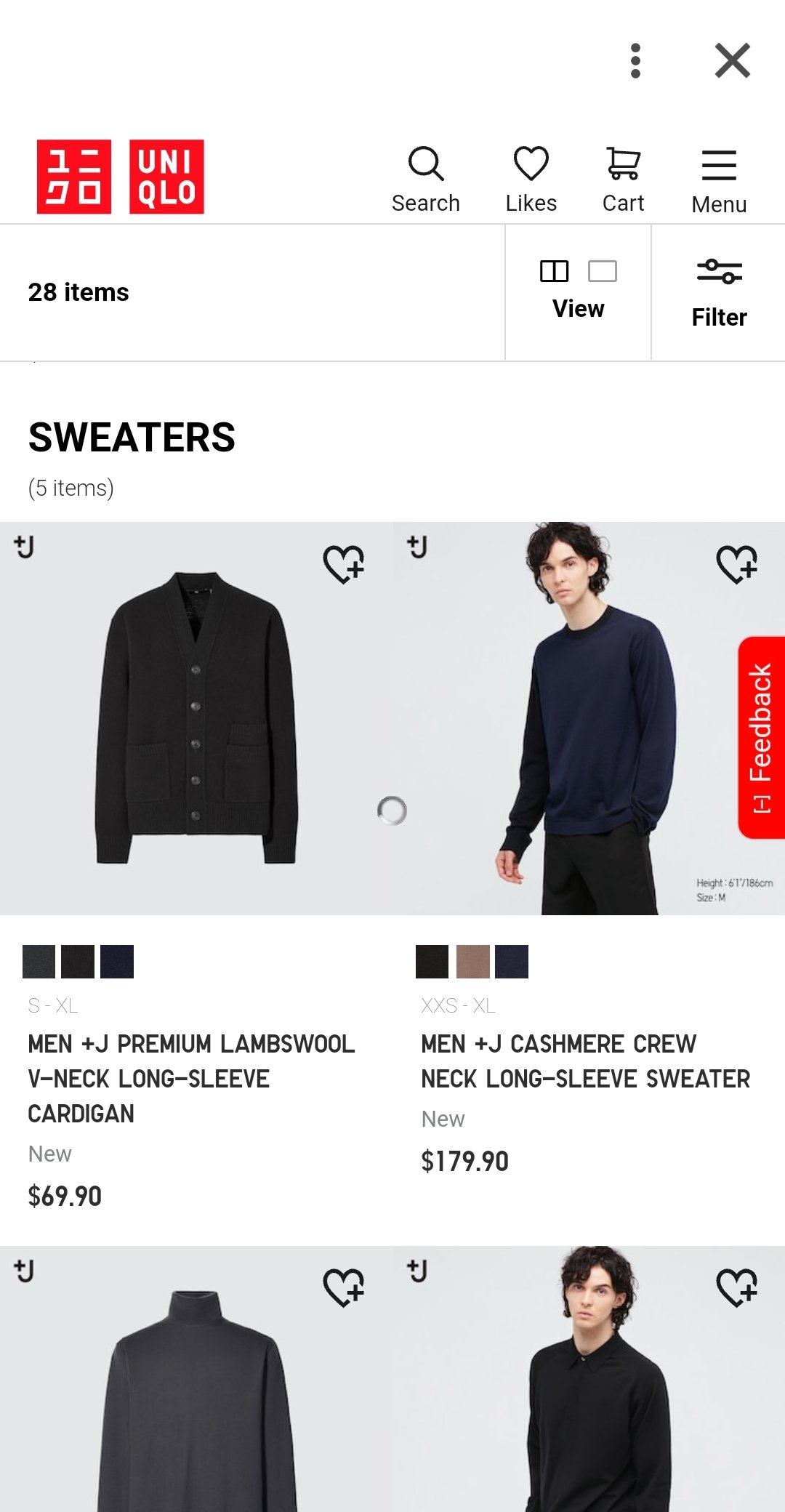Screenshot of a smartphone displaying a shopping page for sweaters from UNIQLO. At the top of the screen, there are three vertical dots on the left and a close button on the right. Below this section, a row of icons features a menu icon, a shopping cart icon, a likes icon, and a search bar. The UNIQLO logo, consisting of two red squares, is situated to the left; one of the squares has text in an unfamiliar language, and the other square displays "UNIQLO."

Underneath the logo, the page indicates that there are 28 items available, with options to change the view (split page or full page) and apply filters. The section header reads "Sweaters – 5 items." The top row displays two photographs of sweaters: 
- On the left, a men's Plus J Premium Lambswool V-Neck Long Sleeve Cardigan is showcased without a model, priced at $69.90.
- On the right, a men's Plus J Cashmere Crew Neck Long Sleeve Sweater is modeled and priced at $179.90.

At the bottom of the page, additional photos illustrate different color variations. One image features a model in a black turtleneck, and another depicts a black button-front shirt.